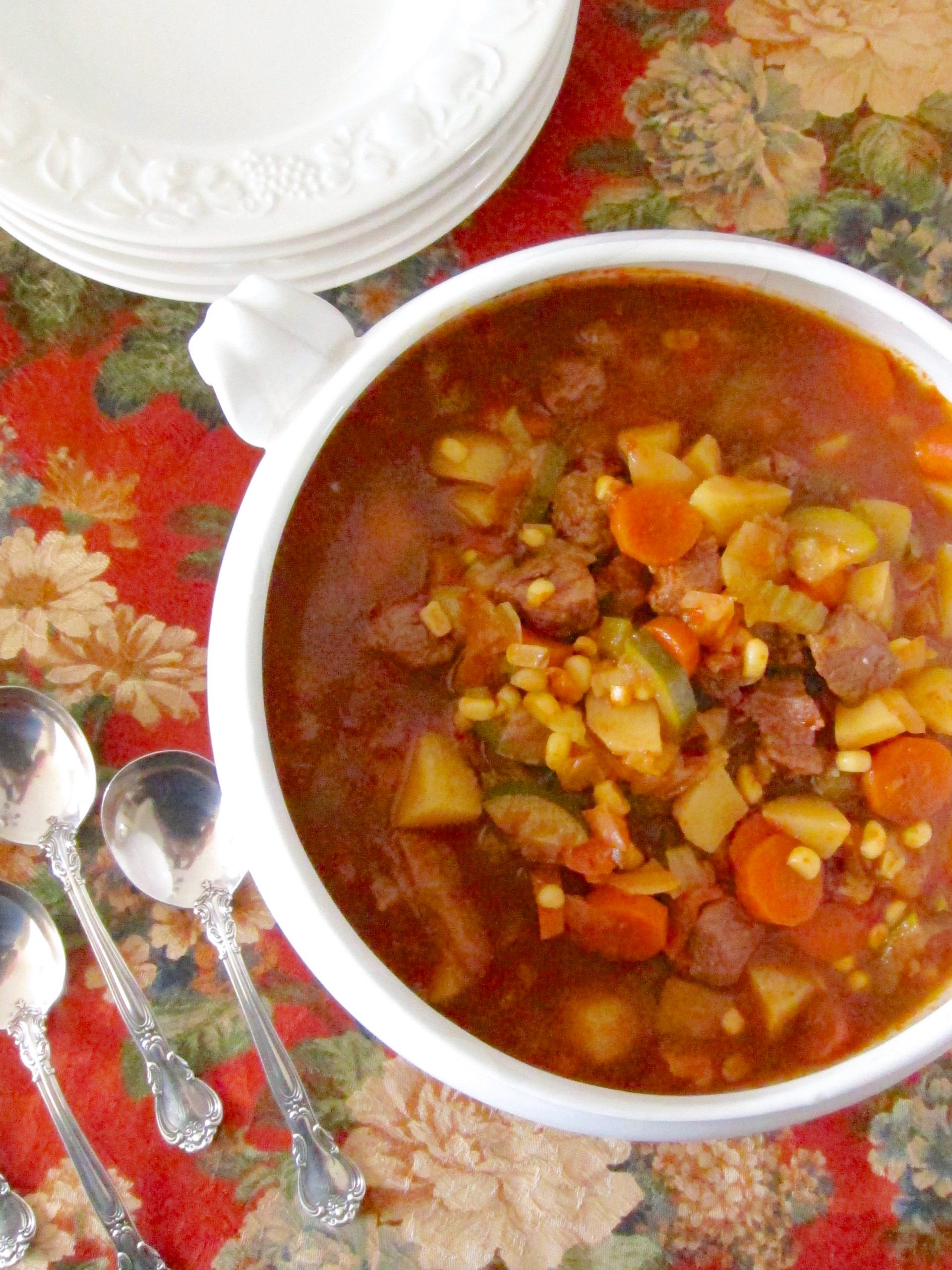This captivating photograph showcases an overhead view of a bowl of rich, reddish-brown soup set on a table adorned with an elegant floral-patterned tablecloth in shades of red, white, green, and yellow. The soup, which appears hearty and inviting, contains a variety of vibrant vegetables such as potatoes, carrots, onions, and corn on the cob, interspersed with chunks of meat. To the left of the soup bowl, elegantly arranged are three silver soup spoons, adding a touch of refinement to the setting. In the corner of the image, partially visible, are multiple stacked white plates with a matching floral design on their rims. The scene is beautifully staged, with no text to distract from the array of colors and the sumptuous meal that takes center stage. The meticulous details of the table setting imply a deliberate and tasteful presentation, evoking a sense of warmth and hospitality.